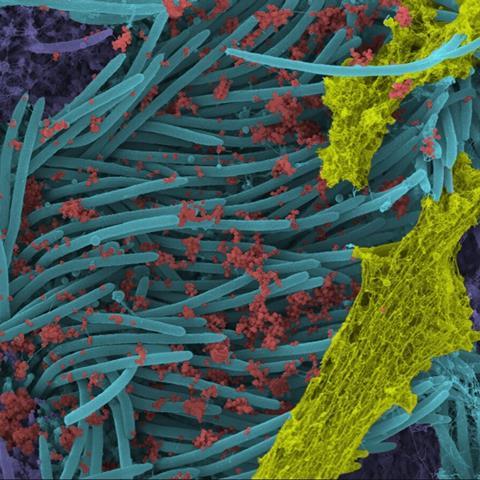The image appears to be a detailed, illustrated depiction of microscopic germs, resembling artwork one might find in a science textbook. Dominating the scene are tentacle-like strips of light blue teal, encircling the entire composition. Interspersed among these tentacles are vibrant red spots, which seem to be scattered randomly across the teal structures. Additionally, thin yellow strands weave throughout, possibly representing mucus or a related substance. Adding to the vivid color palette, purple splotches can be found in the top left, bottom left, and bottom right corners. The overall appearance is reminiscent of a close-up view under a microscope, possibly illustrating bacterial decay or another microscopic phenomenon, with the intricate, colorful details creating a striking and somewhat unusual image.